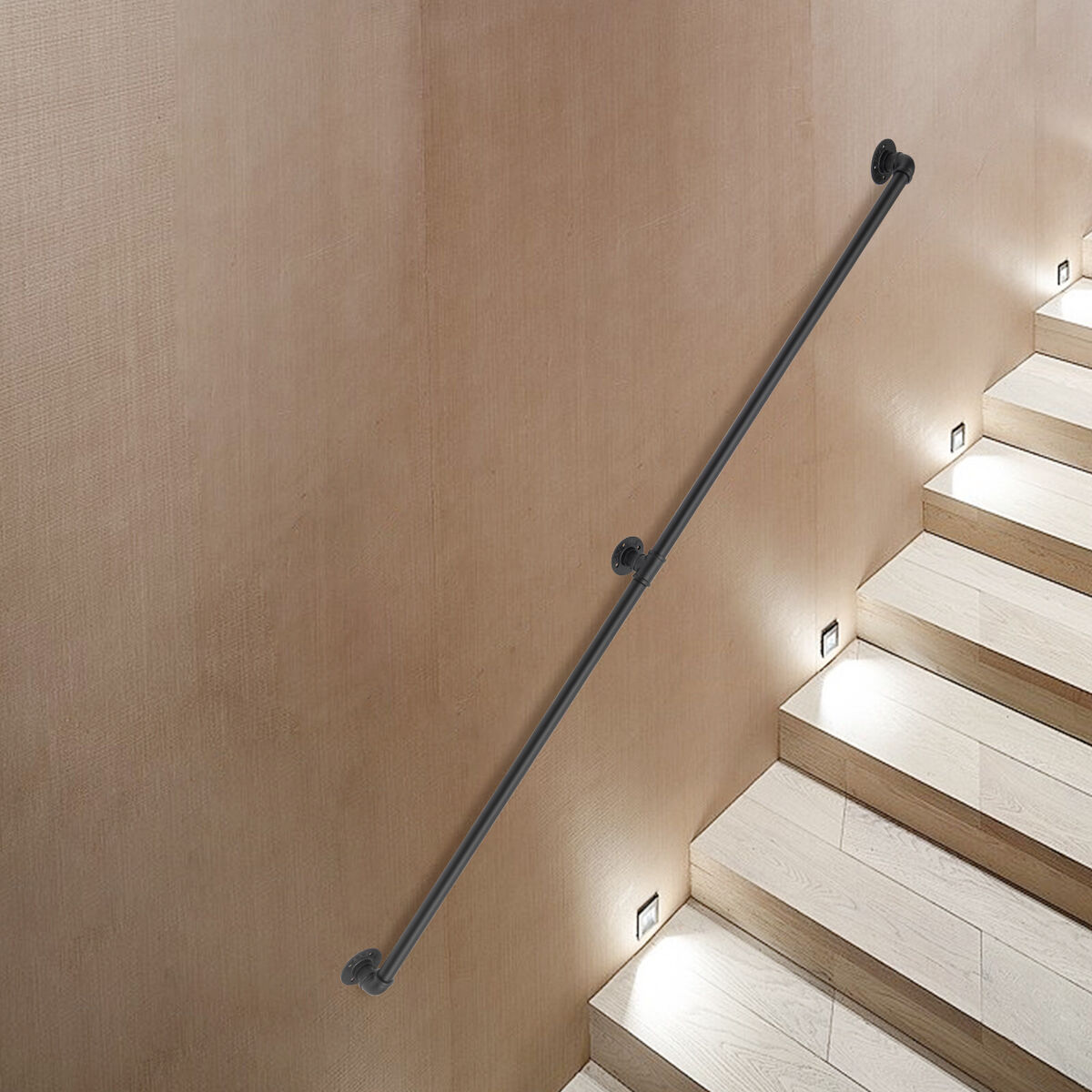The image captures a photograph of a stairwell viewed from an angled perspective, emphasizing its architectural details. The stairwell features neutral tones, with the walls painted a beige color that matches the back of the stair risers. The steps themselves are off-white tiles, uniquely laid out in an asymmetric pattern that diverges from traditional brick or tile arrangements. Each step is illuminated by a series of lights mounted on the risers along the wall, which enhance the brightness of the stair tiles. A black, wrought iron handrail runs diagonally down the wall, attached at three distinct points: at the bottom, middle, and top parts of the visible stairwell section. Despite the angular view, the image clearly highlights the illuminated stair risers, the beige-toned walls, and the distinct design and position of the handrail.